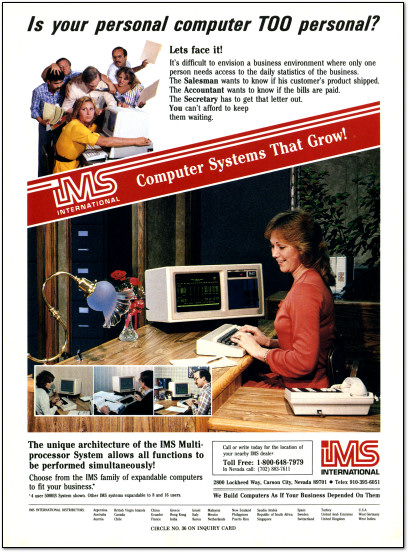The image is an advertisement for IMS International, depicting various elements that underline the utility and collaborative potential of their computer systems. The ad is a small rectangle measuring approximately 4 inches high by 3 inches wide, encased in a thin black pinstripe border, with a slight shadow effect on the right side and underneath. 

At the top, the headline reads, "Is your personal computer too personal?" suggesting the inefficiency of single-user computers in a business environment. Below the headline, text elaborates on the necessity for multiple users to access business statistics, emphasizing various roles such as salesmen, accountants, and secretaries who all require timely information.

The visual center of the advertisement features a woman sitting behind a wooden desk, smiling as she looks down at a piece of paper beside her computer. She is wearing a red shirt and has short brown hair. Her workspace includes a white computer, an adding machine, a curved white lamp, a telephone, and a desk, highlighted in brown.

To the left, there's an illustration of a group of people holding papers and crowding around a computer. A woman, appearing protective, hugs the computer to keep them at bay. Below this scene, a red banner with white text reads, "IMS International Computer Systems that Grow."

Further down, additional paragraphs of text on a white background explain the benefits of the IMS multiprocessor system, which allows simultaneous performance of multiple functions. Three smaller pictures on the lower left show different individuals at their computers, reinforcing the advertisement's message of adaptability and efficiency. Concluding the ad, a block of text encourages potential customers to call toll-free at 1-800-648-7979 to contact IMS International.